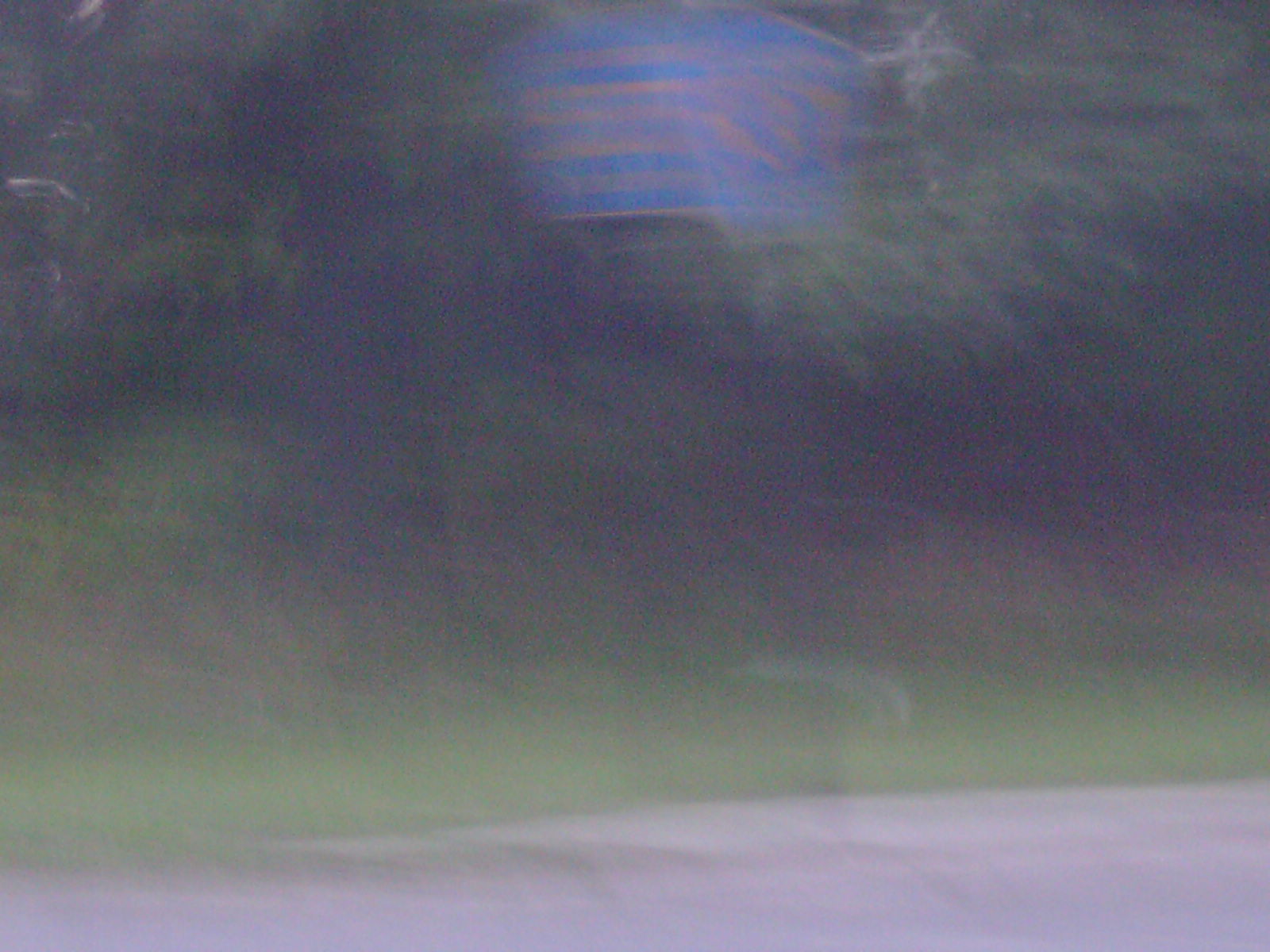This evocative photograph captures an atmospheric, abstract scene dominated by a spectrum of blues, greens, and whites. The bottom portion of the image features a white, horizontal landscape reminiscent of an ethereal terrain. Moving upwards, there appears to be a mid-ground area tinged with green, suggesting the presence of water. The largest section of the photo, occupying the upper expanse, is enveloped in a medium blue haze where the colors seamlessly bleed into each other, creating a dreamy, surreal effect.

Centrally located in the upper part of the image is an intriguing, hexagon-shaped area of brighter blue. This shape is adorned with horizontal, pinkish lines, some of which crisscross, adding to the complexity of the scene. Below this hexagonal figure, wispy clouds drift horizontally, enhancing the sense of layered depth and movement. 

On the left-hand top side of the photo, one can discern subtle streams of wispy, C-shaped clouds that appear to be in gentle motion. The overall composition, with its interplay of colors and shapes, evokes a sense of serenity and intrigue, almost as if one is gazing upon a double-exposed piece of abstract art.